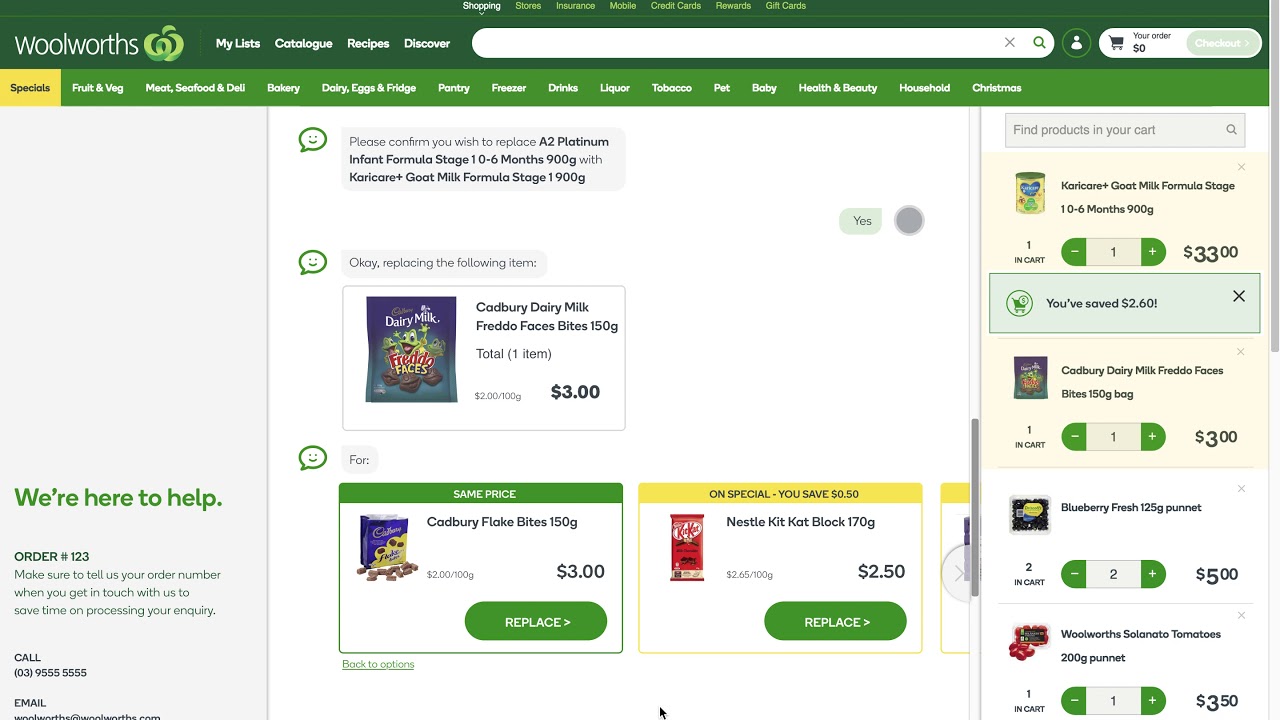This is an image of the Woolworths website. At the top left corner, the Woolworths logo, resembling a green apple, and the website name are prominently displayed. Adjacent to the logo are navigational tabs labelled "My Lists," "Catalog," "Recipes," and "Discover."

To the right of these tabs is a search bar where users can type in queries. Next to the search bar are icons for accessing the user's account and viewing their shopping cart, which currently displays a total of zero dollars. Once items are added to the cart, a checkout button appears.

Below the header, there's a conversational interface, likely with an AI bot. A prompt asks the user to confirm if they wish to replace "A2 Platinum Instant Formula Stage 1, 0-6 months, 900 grams" with "Karicare Goat Milk Formula Stage 1, 900 grams." The user's response is "Yes." The AI bot then confirms, indicating that it will replace the item. It displays a picture and details of the original item, "Cadbury Dairy Milk Freddo Faces Bites 150 grams," priced at three dollars.

The AI bot provides two replacement options: "Cadbury Flake Bites 150 grams" at three dollars, and "Nestle Kit Kat Block 170 grams," which is on special for $2.50 (a savings of 50 cents). Each replacement option has a button allowing the user to confirm the substitution.

On the left side of the webpage, there is a section that reads "We're here to help." Items currently in the shopping cart are displayed on the right side.